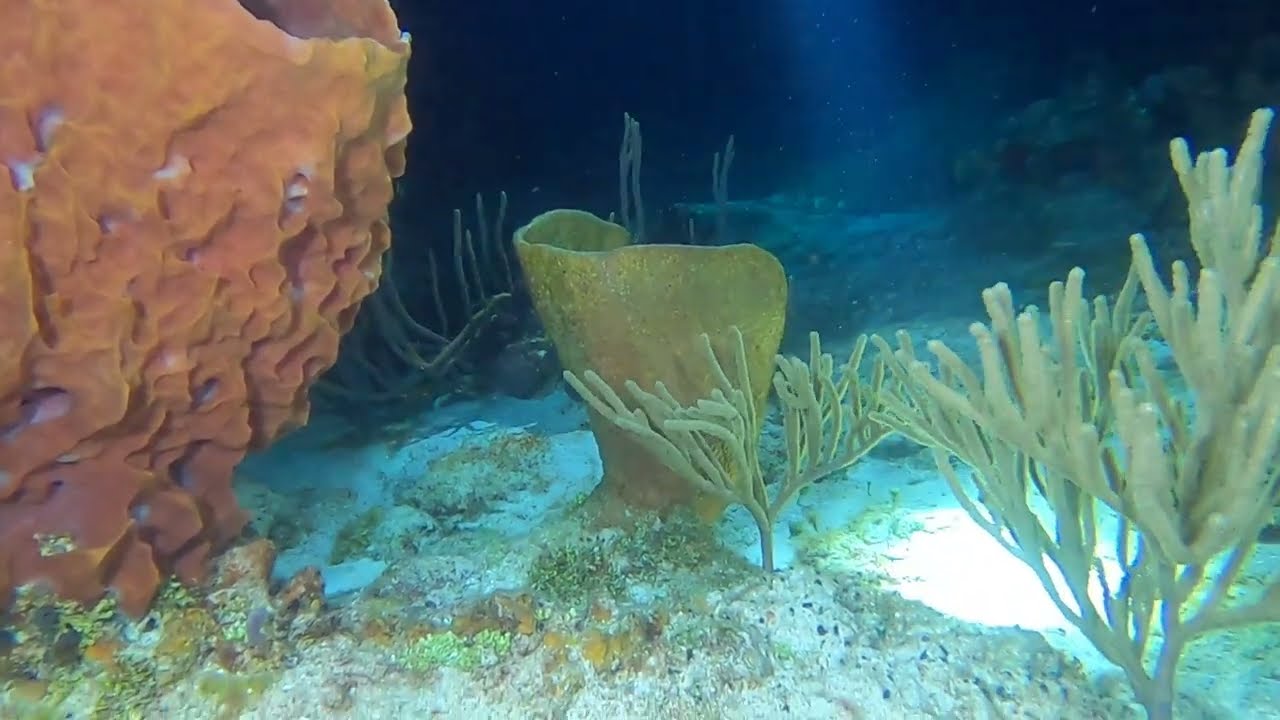This underwater photograph reveals a captivating scene near the ocean floor. The sandy bed is dotted with various organisms and structures, including small vegetation and rock fragments. Central to the image is a prominent orange coral on the left and a yellow vase-shaped coral in the middle. Surrounding them are green, tree-like structures resembling succulents, some of which are further away and blurrier due to the dark background. A bright beam of light penetrates from the surface, illuminating the sandy bottom and accentuating the vibrant colors of the corals and plants. No fish are visible, but the intricate details of the underwater flora create a mesmerizing view of marine life.